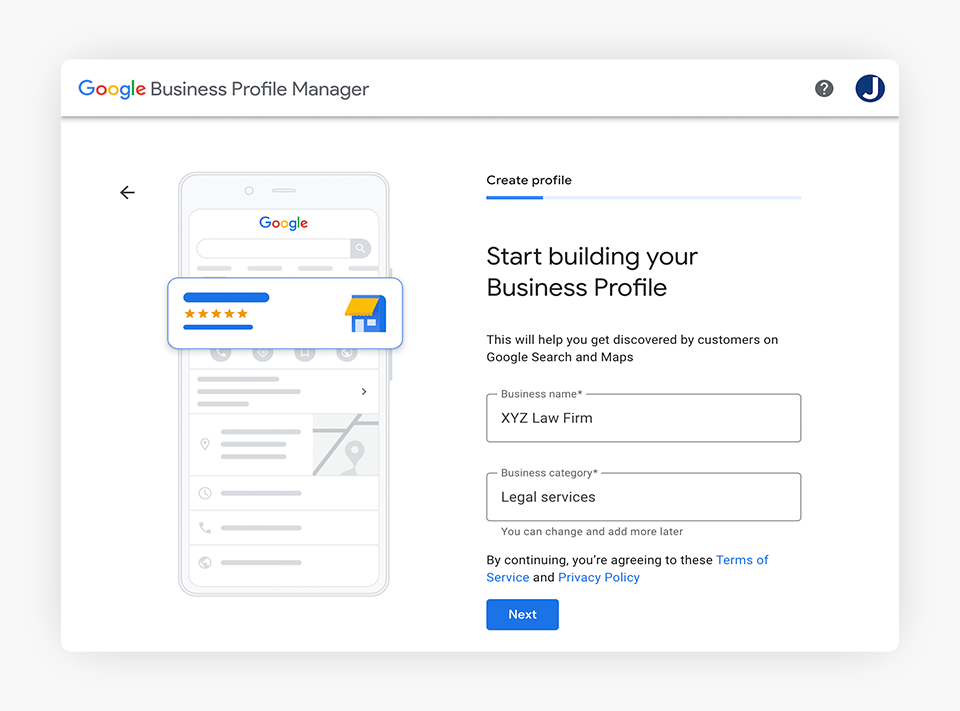The image features a printout set against a light gray background, displaying what appears to be a Google Business Profile Manager page. In the top left corner, there's a question mark inside a gray box and a blue box with a white "J" in it. Directly below these icons, the familiar Google logo is visible, with a blurred-out information box adjacent to it.

At the top right of the printout, the text reads, "Create Profile: Start building your business profile. This will help you get discovered by customers on Google Search and Maps." Below this statement, the form fields include "Business Name," populated with "XYZ Law Firm," and "Business Category," listed as "Legal Services." A note beneath these fields mentions that changes and additions can be made later.

Following this information, a disclaimer states: "By continuing, you're agreeing to these terms," with links to the "Terms of Service" and "Privacy Policy" highlighted in blue. At the bottom of the page, there's a blue box with the word "Next" printed in white. The printout does not contain any further details.